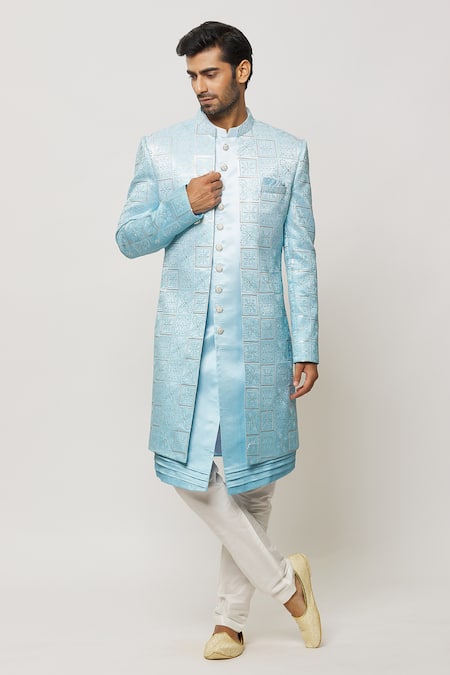In the photograph, a well-groomed man of presumed Asian descent, possibly Indian, stands against a subtle grayish-white background. He has medium, thick, combed black hair and a short, neatly maintained black beard. With his body facing forward and his head turned slightly to the left, he gazes downward. He is dressed in a elegant light blue garment resembling a knee-length silk coat featuring a patterned design and mandarin collar, fastened with buttons down the front. His right hand is raised near his chest, and his left arm rests by his side. Below the coat, he wears form-fitting white pants that extend to the tops of his feet, paired with light ivory or yellowish-white slip-on footwear. His right foot is poised on its tiptoe, crossed over his straight, flat-left leg, evoking a ballet-like posture.